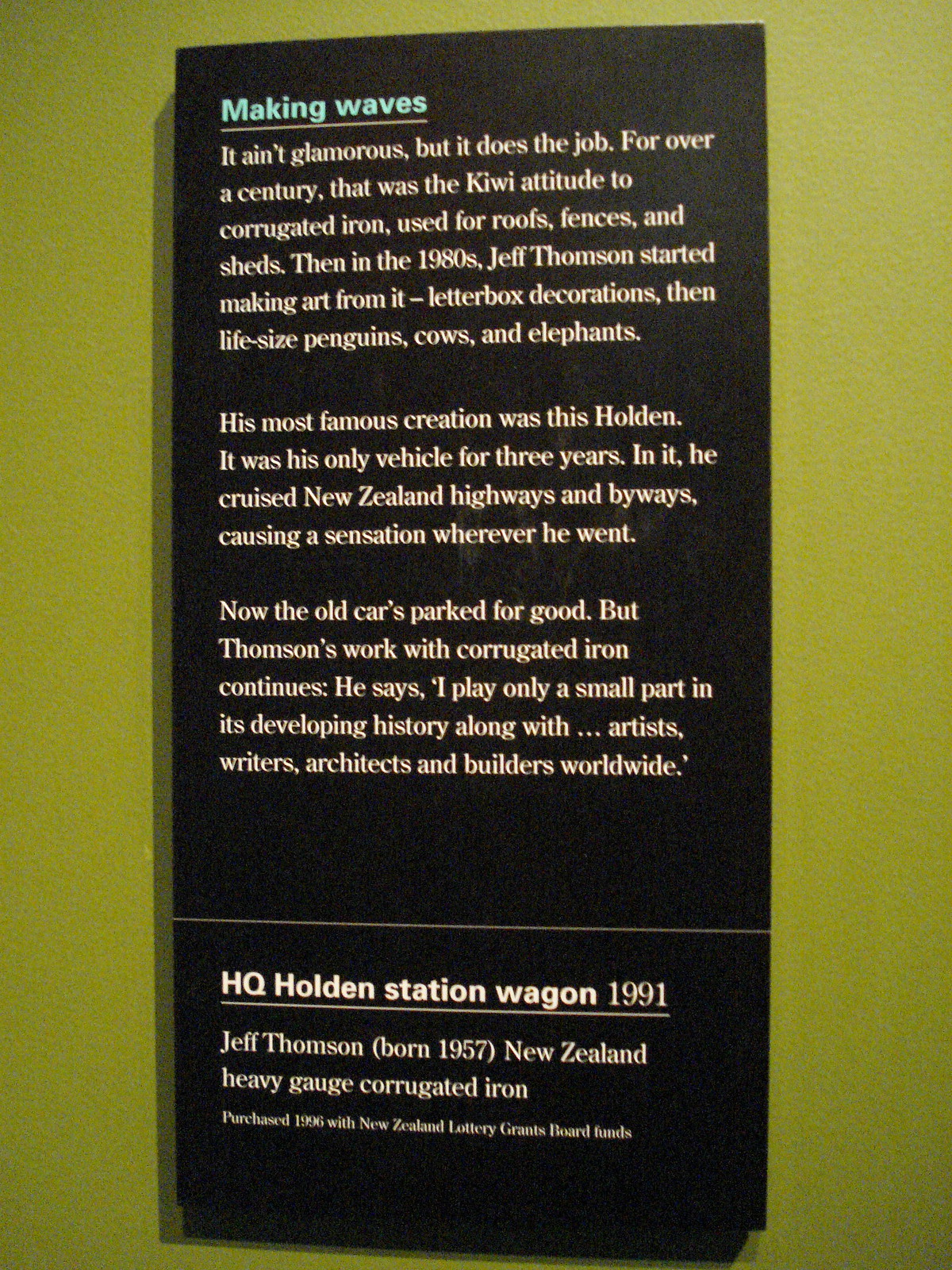The image showcases a museum exhibit sign featuring a detailed description on a black background with white text. The header, written in light blue and underlined, reads "Making Waves". The narrative explains that, although not glamorous, corrugated iron has been relied upon for over a century in New Zealand for roofs, fences, and sheds. The text continues to recount how, in the 1980s, Jeff Thompson transformed this mundane material into art, creating letterboxes, life-sized penguins, cows, and elephants. His standout creation was a Holden station wagon, which he used as his sole vehicle for three years, driving through New Zealand’s highways and byways and captivating the public. Although the vehicle is now retired, Thompson's innovative work with corrugated iron persists. He humbly acknowledges his small contribution to its evolving history among artists, writers, architects, and builders worldwide. At the bottom of the description, it notes, "HQ Holden Station Wagon, 1991" and "Jeff Thompson, born 1957, New Zealand. Heavy gauge corrugated iron". This sign is displayed on a light green wall, adding a subtle contrast to the text.